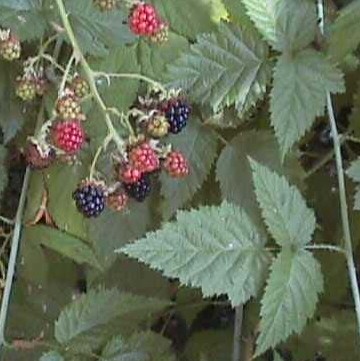This vibrant, square color photograph captures an up-close view of a healthy blackberry bush on a sunny spring day. The focal point of the image is a twig extending from the left side, adorned with an assortment of blackberries and raspberries in various stages of ripeness. Some berries are fully mature and deep black, others are red and still ripening, and several are green and not yet developed. Surrounding the clusters of berries are an abundance of three-sided, jagged-edged leaves that dominate the scene, illustrating the plant's vigorous health. The high level of detail allows the viewer to clearly see the veins within the leaves and the individual segments of each berry. The photograph captures not only the berries and leaves in the foreground but also hints at the lushness of the larger bush in the background.